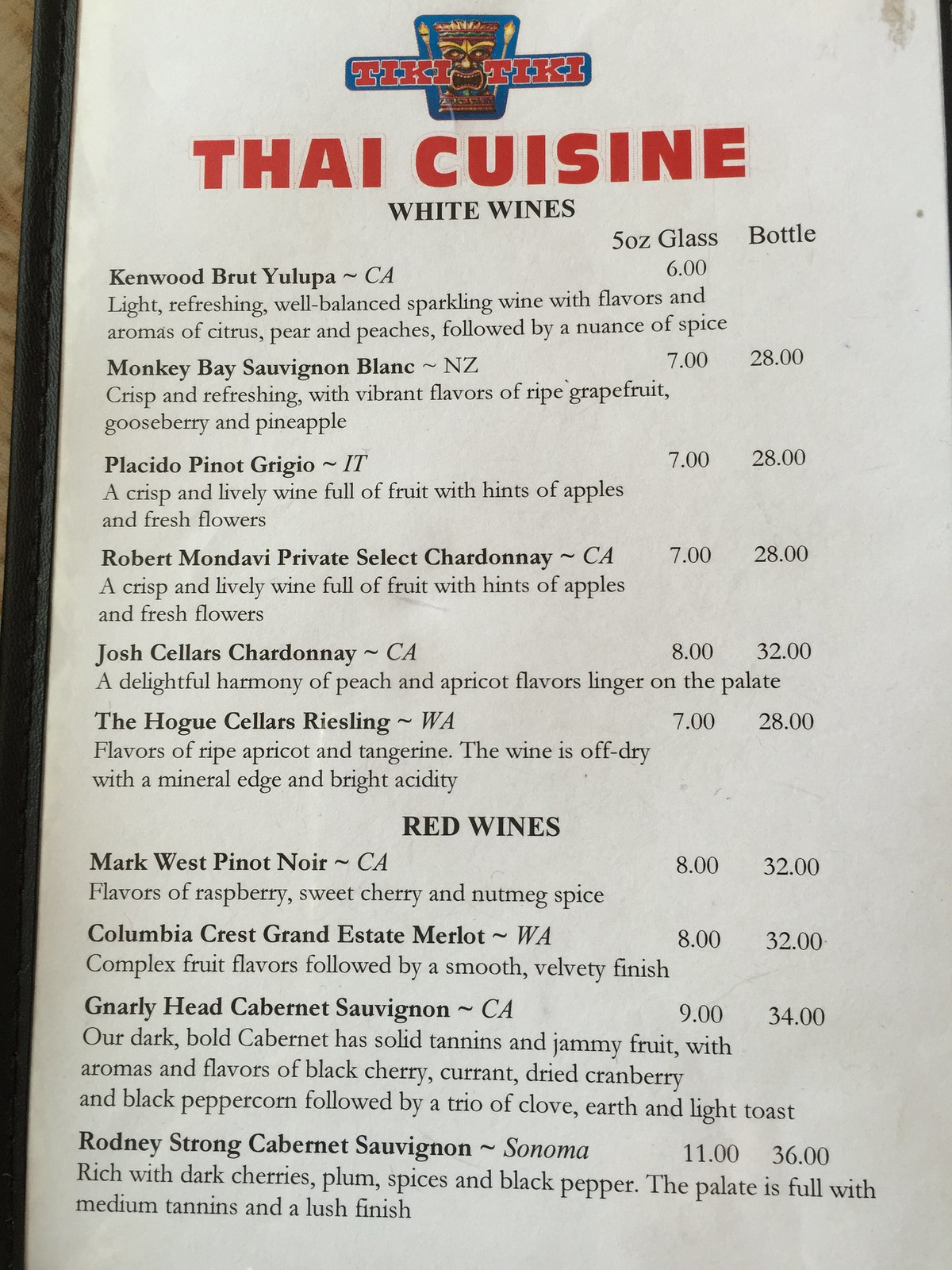This photograph captures a detailed view of a menu from a Thai restaurant, laid flat on a table. At the top of the menu, a tiki symbol and mask graphic are prominently displayed alongside traditional lanterns. The text "Tiki Tiki" is written in bold red letters against a blue background. Below this, the menu headline reads "Thai Cuisines" in large, bold red print.

The menu section featured in the image lists various white wines, each detailed with their origin, available serving sizes, and prices. The list includes:

- **Kenwood Brut Yulupa** (California): $6 for a 5oz glass.
- **Monkey Bay Sauvignon Blanc** (New Zealand): $7 per glass or $28 per bottle.
- **Placido Pinot Grigio** (Italy): $7 per glass or $28 per bottle.
- **Robert Mondavi Private Select Chard** (California): $7 per glass or $28 per bottle.
- **Josh Cellars Chardonnay** (California): $8 per glass or $32 per bottle.
- **Hogue Cellars Riesling** (Washington): $7 per glass or $28 per bottle.
- **Mark West Pinot Noir** (California): $8 per glass or $32 per bottle.
- **Columbia Crest Grand Estates Merlot** (Washington): $8 per glass or $32 per bottle.
- **Gnarly Head Cabernet Sauvignon** (California): $9 per glass or $34 per bottle.

The menu text is primarily printed in black, with detailed information about each wine option, making the selection clear and easy to read.